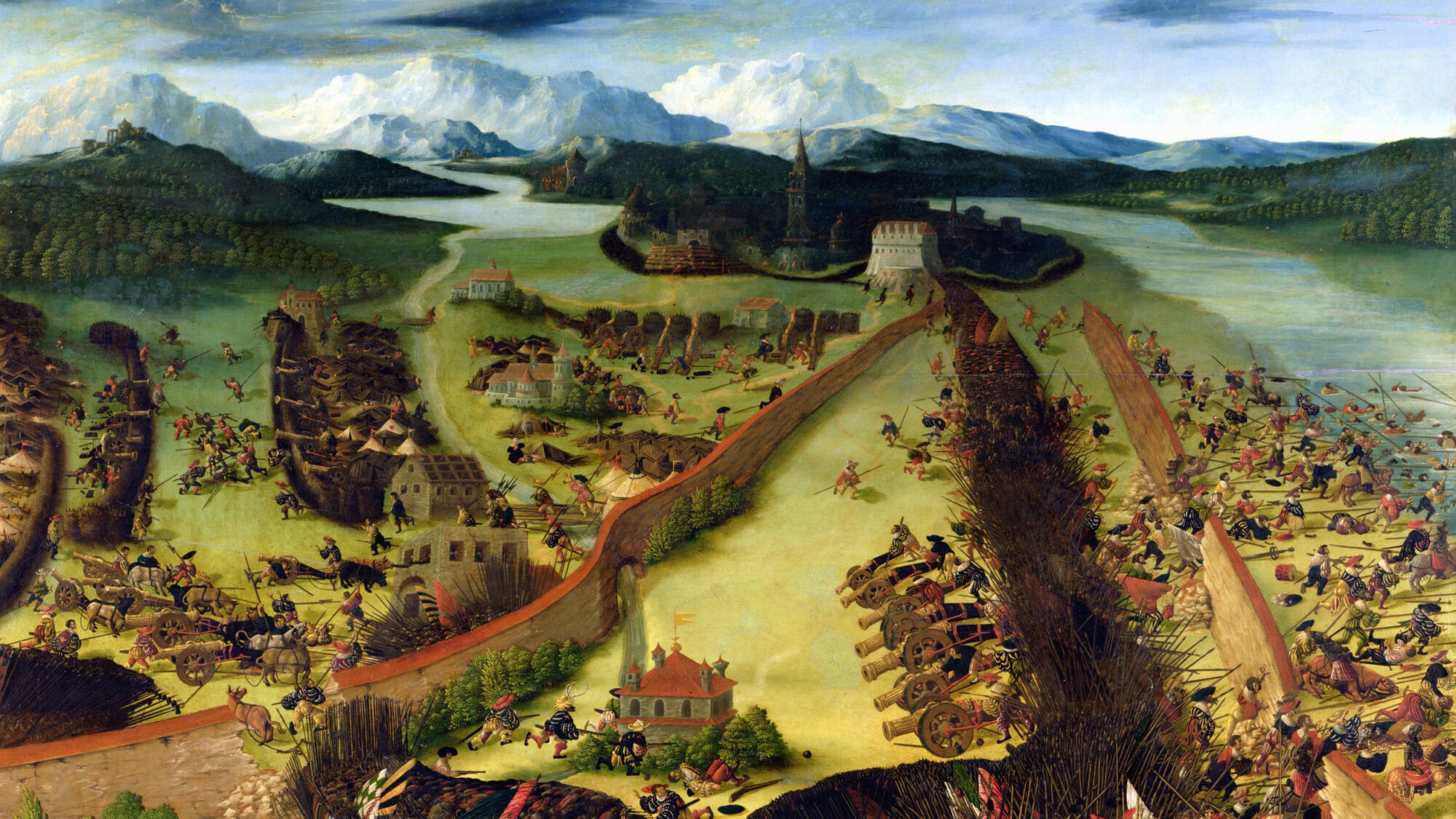This detailed illustration, reminiscent of a painting, depicts an intense battlefield from centuries ago, possibly the 1700s or 1800s. An aerial view reveals soldiers clashing with melee weapons near a fortified structure with multiple defensive layers. The initial confrontation occurs by a tall brick wall on the right, where the fighters have breached a second barricade made of stacked sticks. Alongside, cannons with large wheels are strategically placed. As the battle extends towards a large river running beside the estate, combatants are seen fighting on the shore and even in the water. The scene is rich with historical buildings, including homes and a church, surrounded by soaring, snow-covered mountains under a blue sky. Notably, there are also big wooden ships depicted near additional fortifications and shrubbery barriers, adding to the grandiosity and chaos of the depicted warfare.